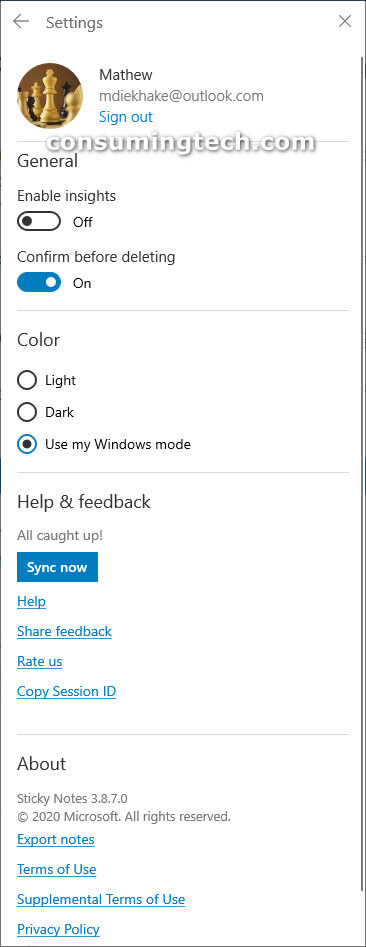This is a screenshot of the settings menu in Microsoft Sticky Notes. The background is white at the top, with gray font displaying the word "Settings." In the upper right corner, there is an "X" button to close the pop-up menu, and on the upper left, an arrow pointing to the previous menu.

Below the header, there's a profile section featuring a profile picture depicting a white queen on a chessboard, followed by the username "Matthew" and the email "m****@outlook.com." There's also a blue "Sign out" link beneath the email. A watermark reading "consumingtech.com" in white bubble letters overlays the image.

In the "General" section, the first option is "Enable insights," with a toggle button set to "Off." The next option is "Confirm before deleting," with a toggle button set to "On," highlighted in blue. Further down, there's a "Color" section with options for "Light," "Dark," or "Use my window mode," with the latter selected by Matthew. At the bottom of the menu, the "Help and Feedback" section indicates "All caught up."